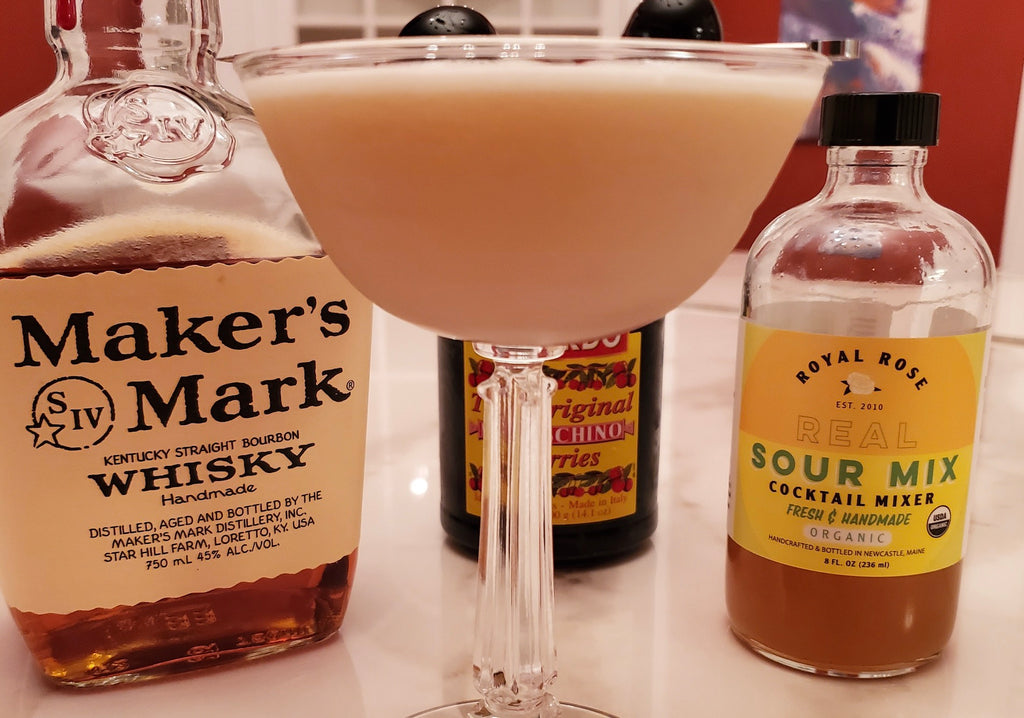This image features a detailed arrangement of cocktail ingredients and a prepared drink placed on a table covered in a white cloth. Dominating the center of the photo is a tall glass filled with a pale beige cocktail. To the left, there's a clear bottle of Maker's Mark Kentucky Straight Bourbon Whiskey, noticeable by its peach-colored label with black lettering that reads "Maker's Mark Handmade." Behind the cocktail glass, a jar of maraschino cherries is partially visible, displaying fragments of the words "Chino," "original," and "Rees" on its label. On the right side of the table, there's a bottle of Royal Rose Sour Mix. Its label is orange and yellow with black and green lettering indicating it is a "Fresh and Handmade Organic Cocktail Mixer." The background features a red and white colored wall, with a painting on the right side that's not entirely discernible.